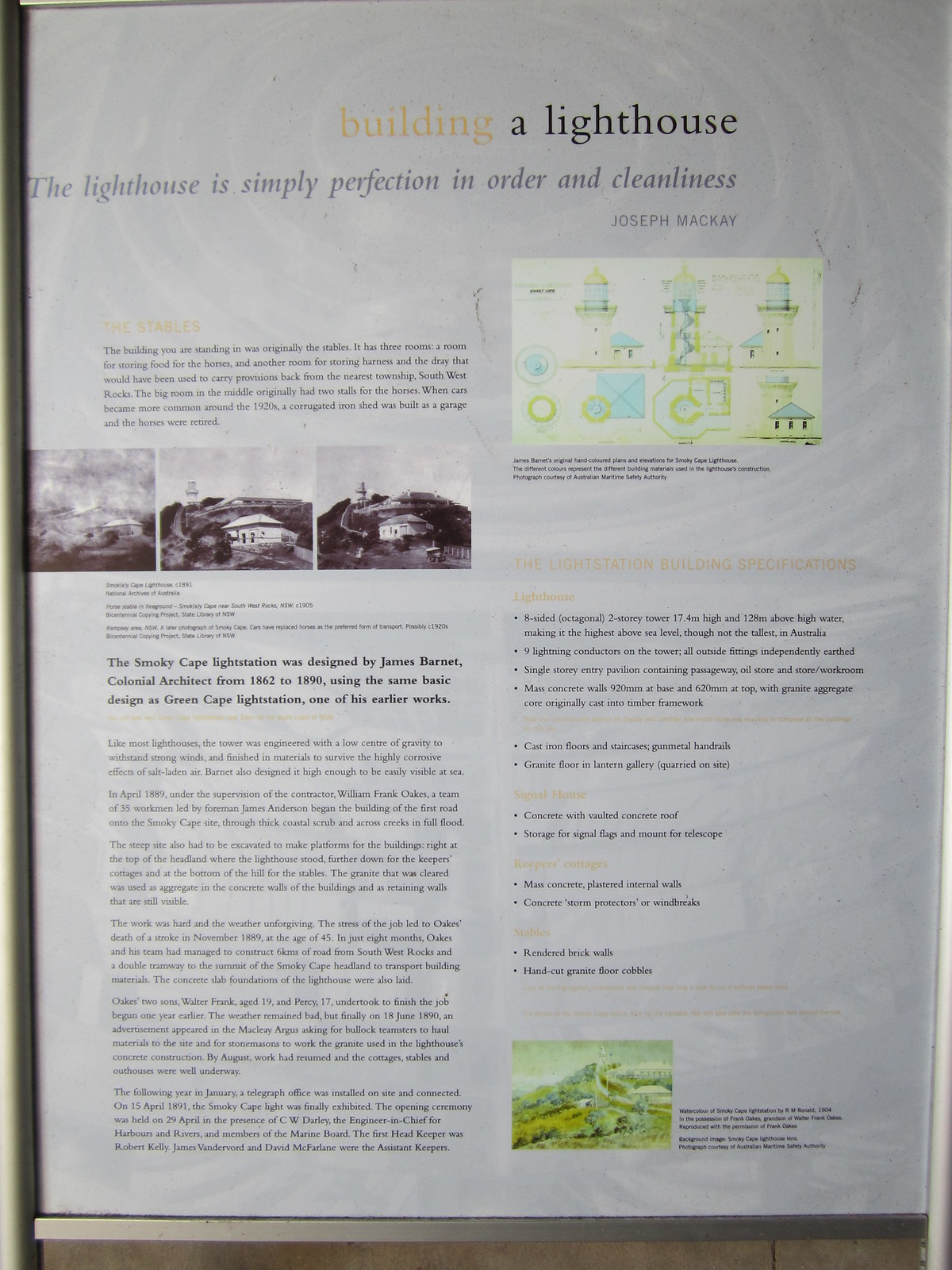The image is a detailed informational display, resembling a museum plaque or signage, primarily with an off-white background. At the top, the centered title reads "Building a Lighthouse," where "Building" is in light yellow and "a lighthouse" is in black. Below the title in smaller, gray italic text, it says, "The lighthouse is simply perfection in order and cleanliness," attributed to Joseph McKay in all caps and slightly smaller, straight-aligned black text.

The display is divided into two main columns. The left column features several black-and-white photographs arranged in a row, each depicting what appears to be a one-story house or building, collectively occupying less than 10% of the column's height. Similarly, an array of small, less legible paragraphs is positioned throughout the column, adding historical context.

On the right column, a colorful map in blue, green, and white provides additional spatial orientation. Architectural drawings of the lighthouse appear at the top right, followed by text detailing the specifications of the light station building. Information is provided about the design by James Barnett, a colonial architect, noting that the Smoky Cape Light Station follows the same design principles as his earlier work, the Green Cape Light Station. At the bottom right, a color photograph offers a scenic view of the area surrounding the lighthouse, complementing the historical narrative and visual documentation provided throughout the display.